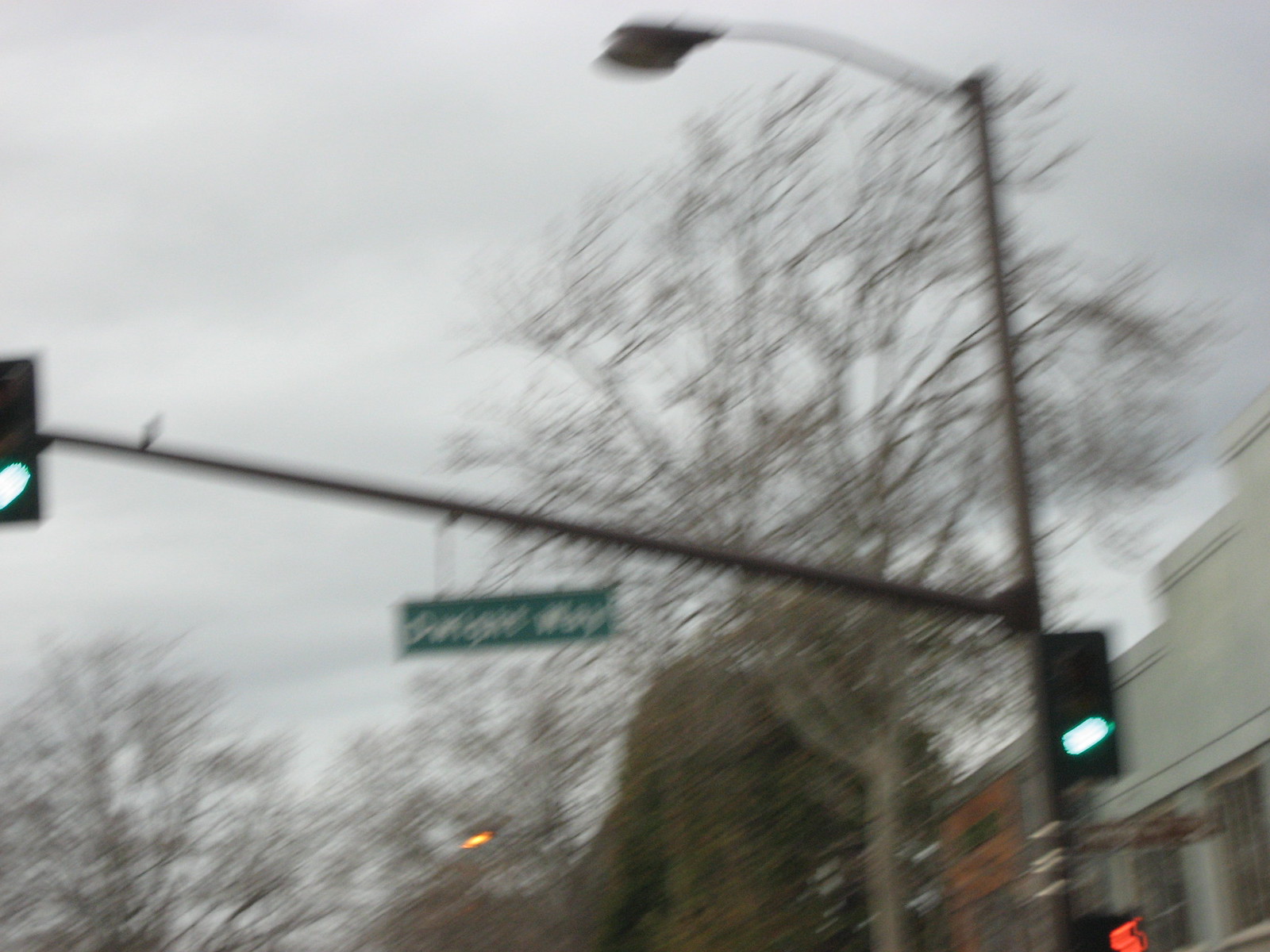In this blurry photograph taken during the day, a cloudy, possibly rainy sky looms overhead, painting a gloomy, gray ambiance. The scene captures a street view characterized by a tall black street light extending to the left, crowned with a green traffic light. Midway along the horizontal pole, a green street sign with white lettering hangs down, although its text is obscured by the photo's lack of clarity.

Adjacent to the street light, there is a smaller crossing sign positioned lower on the post, seemingly glowing red through the haze. To the right, the tops of several buildings, one gray and another with a red brick facade, are visible amidst bare trees that stretch across the frame, suggesting a chilly, wintry day. The overall scene evokes a dreary, overcast day, marked by indistinct details due to the photo's blurriness.